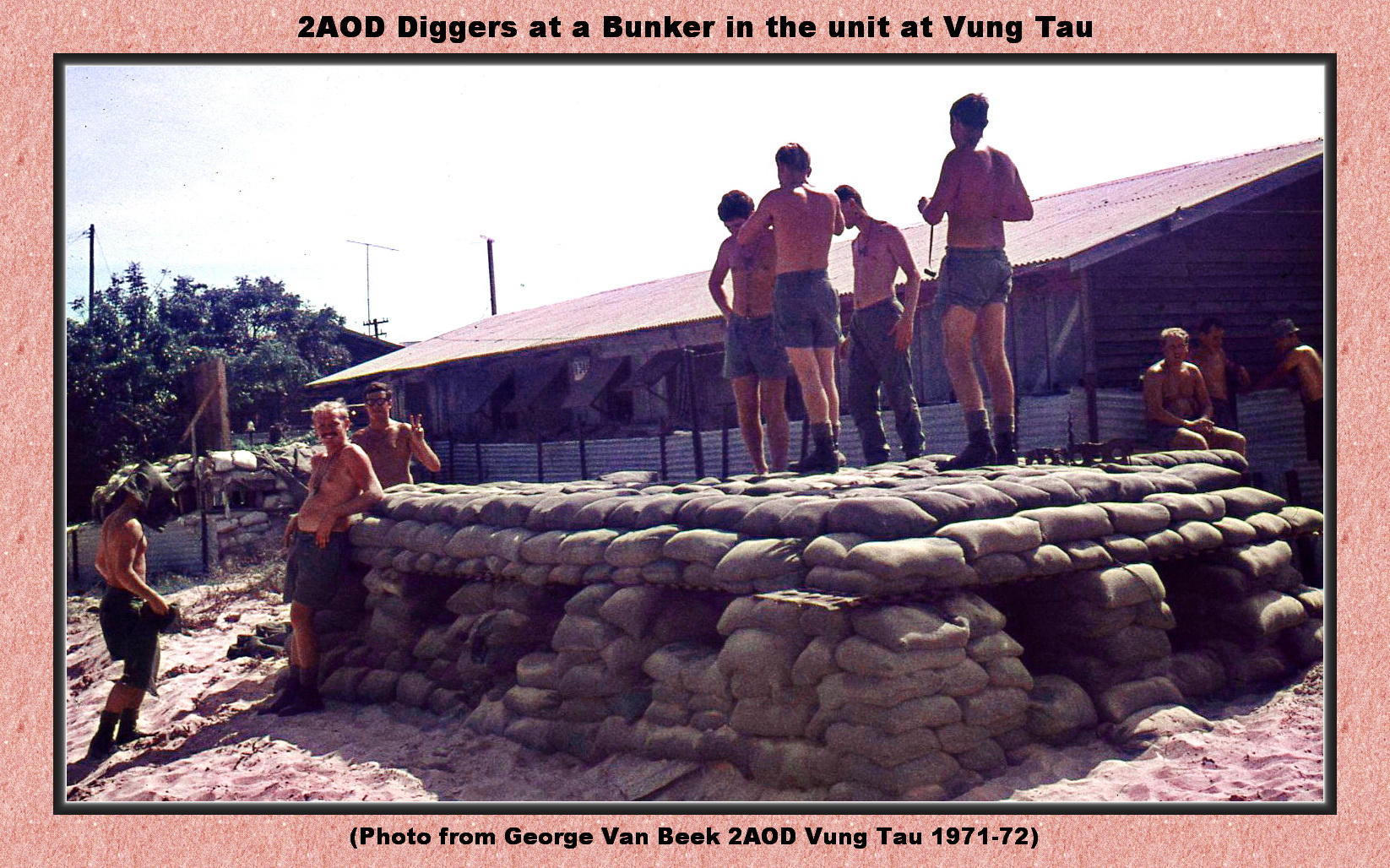The image displays a rectangular photograph taken outdoors during the daytime, framed by a gradient pink sandstone border. At the top of the border, bold black text reads, "Two A.O.D. Diggers at a Bunker in the Unit in Vung Tau," and at the bottom, a caption within parentheses notes, "Photo from George Van Beek, Two A.O.D. Vung Tau, 1971-72."

The central focus is a bunker constructed from stacked sandbags, rising around four layers high, with additional layers forming a roof. On top of the bunker, four shirtless, tanned men of Caucasian descent are positioned; three wear jean shorts while the fourth wears long jeans. Most of these men are shoeless, except for one. One man stands to the left of the bunker, another leans against it, and two men are stationed behind it. One individual in the back-left corner smiles and looks at the camera, while another behind him, sporting glasses, flashes a peace sign. The sky above is a grayish-white.

In the background, there's a long row of houses with slanted roofs, constructed from wood and sheet metal, and to the left of the scene, some trees are visible, enhancing the outdoor setting’s authenticity.